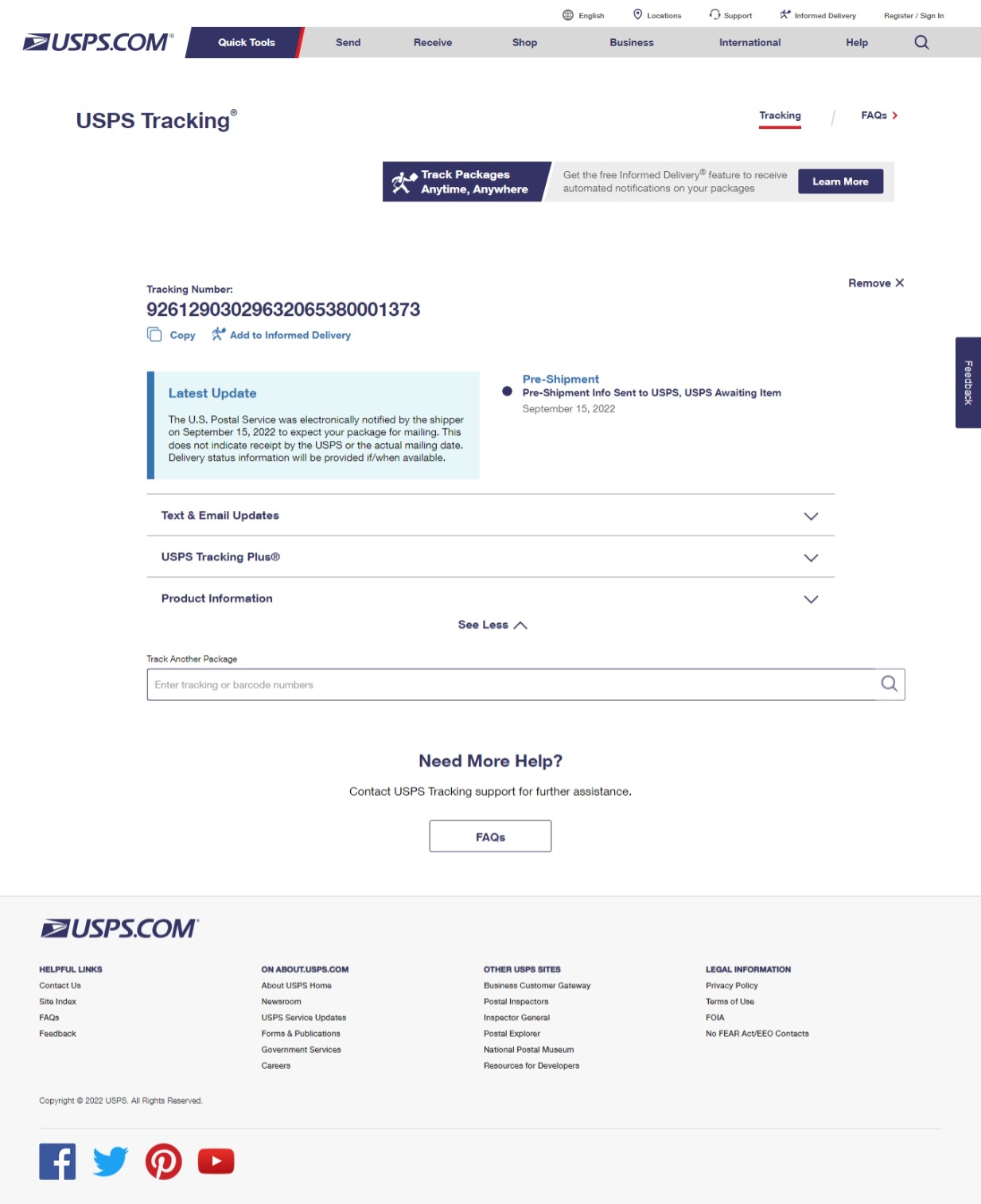In this detailed screenshot of a USPS tracking page, the viewer's attention first lands on the prominent elements at the top left, starting with the iconic blue USPS logo followed by "USPS.com." The page's navigation menu includes toolbars with several options: "Quick Tools" highlighted in blue with a red underline, and additional options in gray—"Send," "Receive," "Shop," "Business," "International," "Help," and a search bar for user convenience.

Above the toolbars, there are more headers for site functions, such as "English Location," "Support," "Informed Delivery," "Register," and "Sign In." Below, on the left side, the section labeled "USPS Tracking" is distinguished by a copyright symbol and a red underline. Nearby is a clickable "Fax" option marked with an arrow.

The left-hand side features a gray toolbar emphasized by a blue highlight, illustrating a man carrying baggage. It touts the benefits of "Track packages anytime, anywhere" and promotes the "Free Informed Delivery" feature for automated package notifications, accompanied by a blue "Learn More" link.

Central to the page is the primary focus: the tracking number, displayed boldly in blue. The number reads "926-1290-3029 632-065-3800 1373" with options to "Copy" or "Add to Informed Delivery" available in blue text.

Directly below, a light blue informational box titled "Latest Update" conveys: "US Postal Service was electronically notified by the shipper on September 15, 2022, to expect your package for mailing. This does not indicate receipt by USPS or the actual mailing date. Delivery status information will be provided when available."

To the right, the "Pre-Shipment" section details: "Pre-Shipment Info for USPS. USPS Awaiting Item, September 15, 2022." Below, there are dropdown options for "Text and Email Updates," "USPS Tracking Plus," and "Product Information," alongside a "Show List" to manage tracking.

For further action, users can "Track Another Package" by entering additional tracking or barcode numbers. Assistance options include a notice reading "Need more help? Contact USPS for further assistance," alongside a "Fax" square.

At the bottom of the page, viewers find icons for social media platforms—Facebook, Twitter, Pinterest, YouTube—alongside multiple clickable links for additional resources and information.